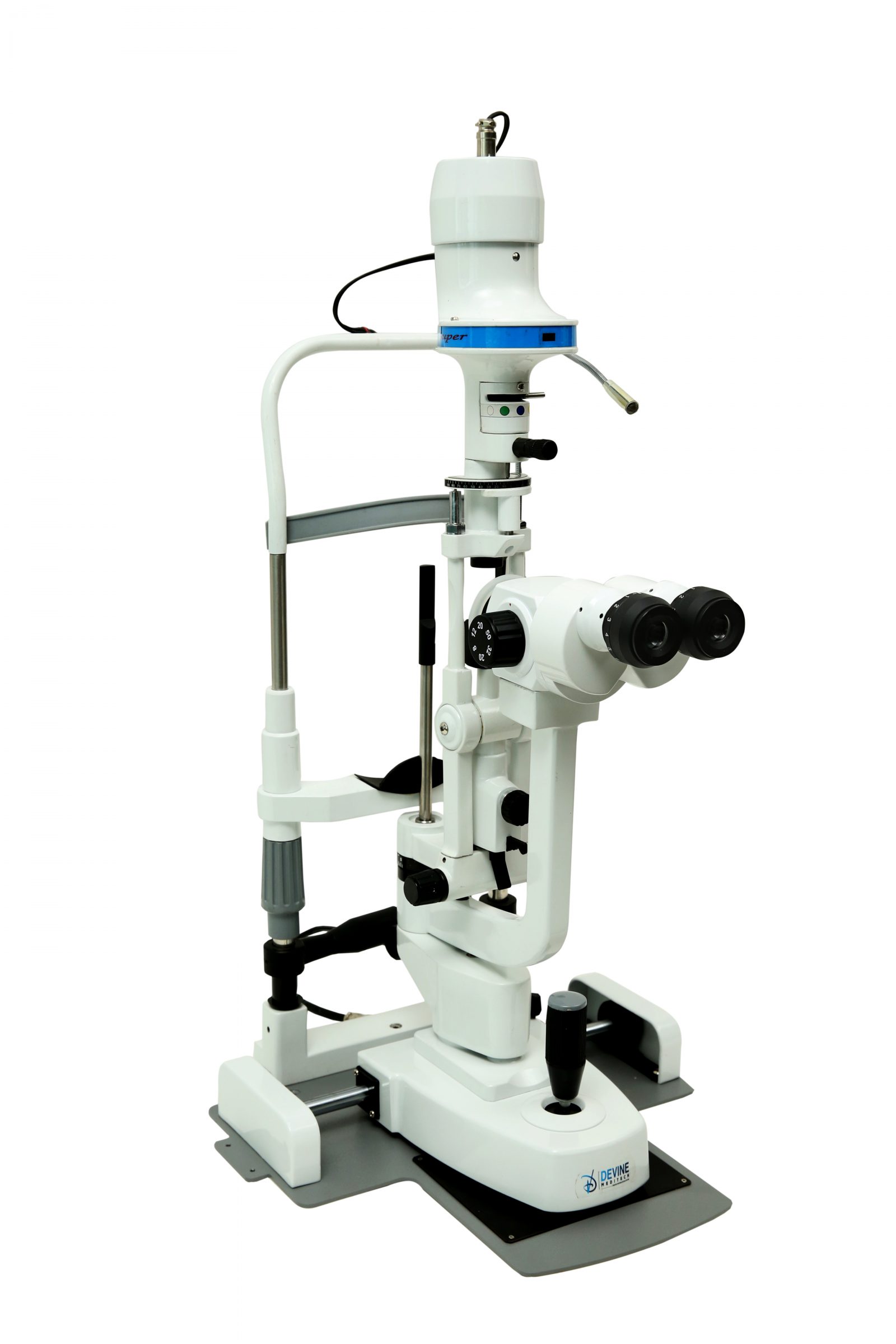The image depicts a tall, advanced optometry device, primarily white in color, with a sleek, modern design. It features a pair of black binocular-like eyepieces situated on the right, giving it a microscope-like appearance. The device has a cylindrical top with a blue rim, leading down to various dials and mechanisms, including an adjustable black part at the front. A notable component is the joystick at the base, used for precise adjustments. Additionally, there's a grey forehead strap and a chin rest on the far side, indicative of its usage in eye examinations. The device bears the logo "Divine" in blue, positioned prominently on the front. The background is white, accentuating the device's clean and professional aesthetic.